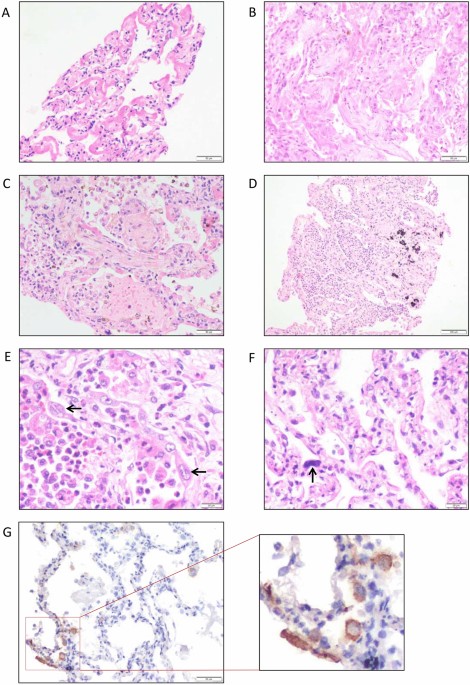The image consists of eight panels, arranged in two columns of four images each, depicting a series of microscopic views of what appear to be biological samples, likely of human origin. Panels A through F primarily feature cells stained in various shades of purple against a white background. 

- **Panel A** displays a triangular cluster of purple cells with numerous black dots, oriented from the bottom left to the top right. 
- **Panel B** is densely packed with purple cells lacking black dots.
- **Panel C** resembles Panel A but is less vibrant, appearing more pink with many black dots, and oriented from the top left to the bottom right.
- **Panel D** contains a few black blotches on the right side, forming a shape reminiscent of a heart, sharing the same faded pink hue as Panel C.
- **Panel E** returns to the more vivid purple cells found in Panels A and B, though it's scattered with darker purple dots and has few black dots.
- **Panel F** showcases a series of purple squiggles with deep purple dots. 

Panel G, distinguished by its blue and orange (or brown) staining, stands out and includes two arrows pointing from the lower left-hand corner to an adjacent, unlabeled inset panel. The inset provides a magnified close-up of the cells in Panel G, revealing them in more detail with brown, black, and blue features. Each panel is outlined in black, emphasizing the detailed observation of the biological specimens.